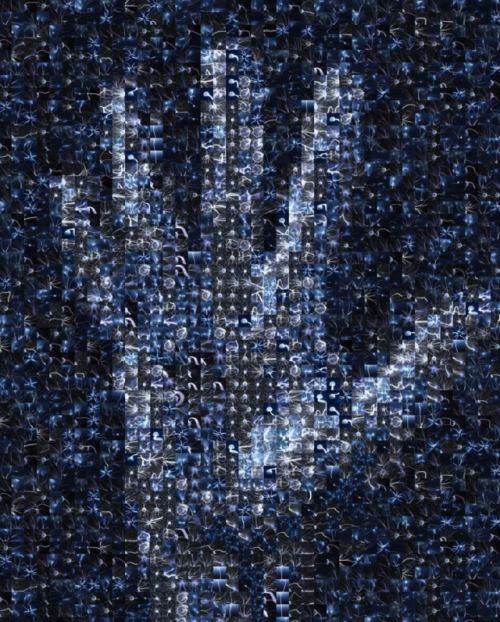This image depicts a computer-generated artwork or possibly a painting, featuring an abstract representation of a human hand. The artwork itself is vertically rectangular, with no defined borders, and is entirely composed of varying shades of black, blue, and white pixels or squares. The central focal point of the image is a lighter area in the shape of a human hand, with the thumb positioned to the right. This hand extends from slightly below the wrist to just above the fingertips, and its palm is facing the viewer. The hand is constructed from lighter shades of gray and blue, making it stand out against the darker, more saturated background. The background, filled with low-opacity pixels and squares of darker blacks and blues, creates a striking contrast against the hand. Throughout the entire image, there are numerous small, squiggly forms that resemble sperm and eggs, adding a dynamic and intricate texture to the composition.